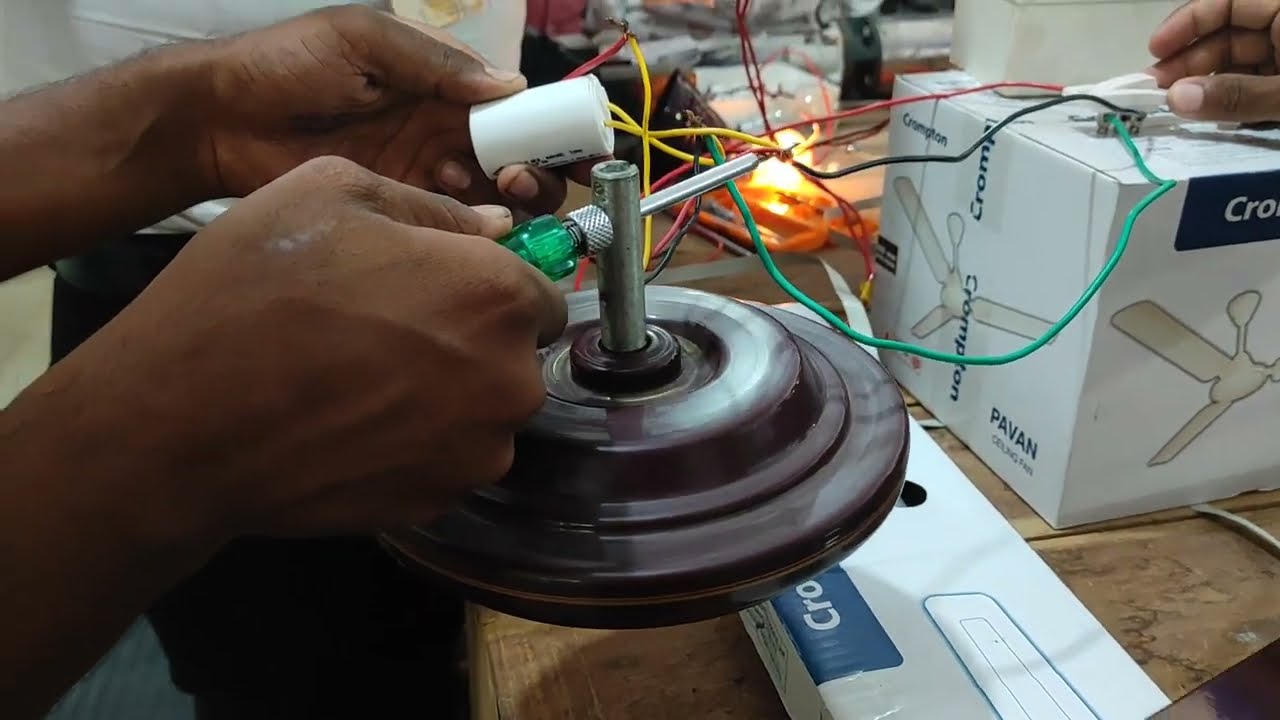In this detailed photograph, we see a close-up of a man with dark skin working meticulously on the base and electronic components of a ceiling fan. His hands and wrists emerge from the left side of the image. In his right hand, he holds a green-handled screwdriver that is threaded through a metal pipe, which is part of the fan's base assembly. His left hand grips a white cylindrical object from which yellow, red, and green electrical wires protrude.

These wires extend towards the upper right corner of the image and connect to another brown-skinned hand, likely belonging to another individual, which is securing a white clamp onto a portion of the wires. The work is being conducted over a cluttered wooden table scattered with various tools and instruments, including a rectangular box nestled beneath the circular base of the fan.

In the background, we see a product box featuring the image and brand of the ceiling fan, Pavan (spelled P-A-V-A-N). The detailed, high-definition photograph's widescreen aspect ratio captures the intricate assembly process and the collaborative effort to piece together the ceiling fan.